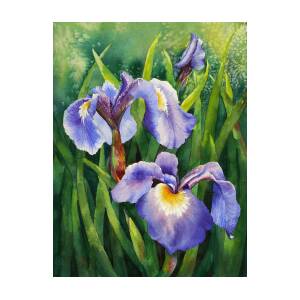The painting features a trio of purple-blue irises with intricate yellow-orange centers. Each iris is painted from a different angle, with one seemingly still in the early stages of blooming. They are surrounded by tall, luscious blades of grass that evoke a green bean-like appearance, creating a rich, textured foreground. The petals of the irises are intentionally droopy, curving outward as if wilting, adding a touch of melancholy to their delicate beauty. Behind the flowers stretches a hazy, lime-green background that heightens the vibrant greens of the grass and gives a sense of depth. There is no visible artist's signature on the piece. The contrast between the vivid green grass and the serene irises coupled with their detailed centers, which transition from yellow to a more orange hue, captures a close-up, intimate moment in this imagined landscape.